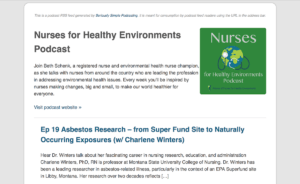The image appears to be a cropped screenshot from an article section of a website. At the top of the image, there is a title that reads "Nurses for Healthy Environments Podcast," but the text is quite small and hard to decipher. Beneath this title, there seems to be a paragraph providing a description, though the text is not clearly visible in the image. On the right side of the image, there is a prominent green box. At the top of this box, the word "Nurses" is displayed, accompanied by a white globe icon. Below this, in blue text, it reads "Episode 19: Asbestos Research - From Superfund Site to Naturally Occurring Exposures with Charlene Winters."